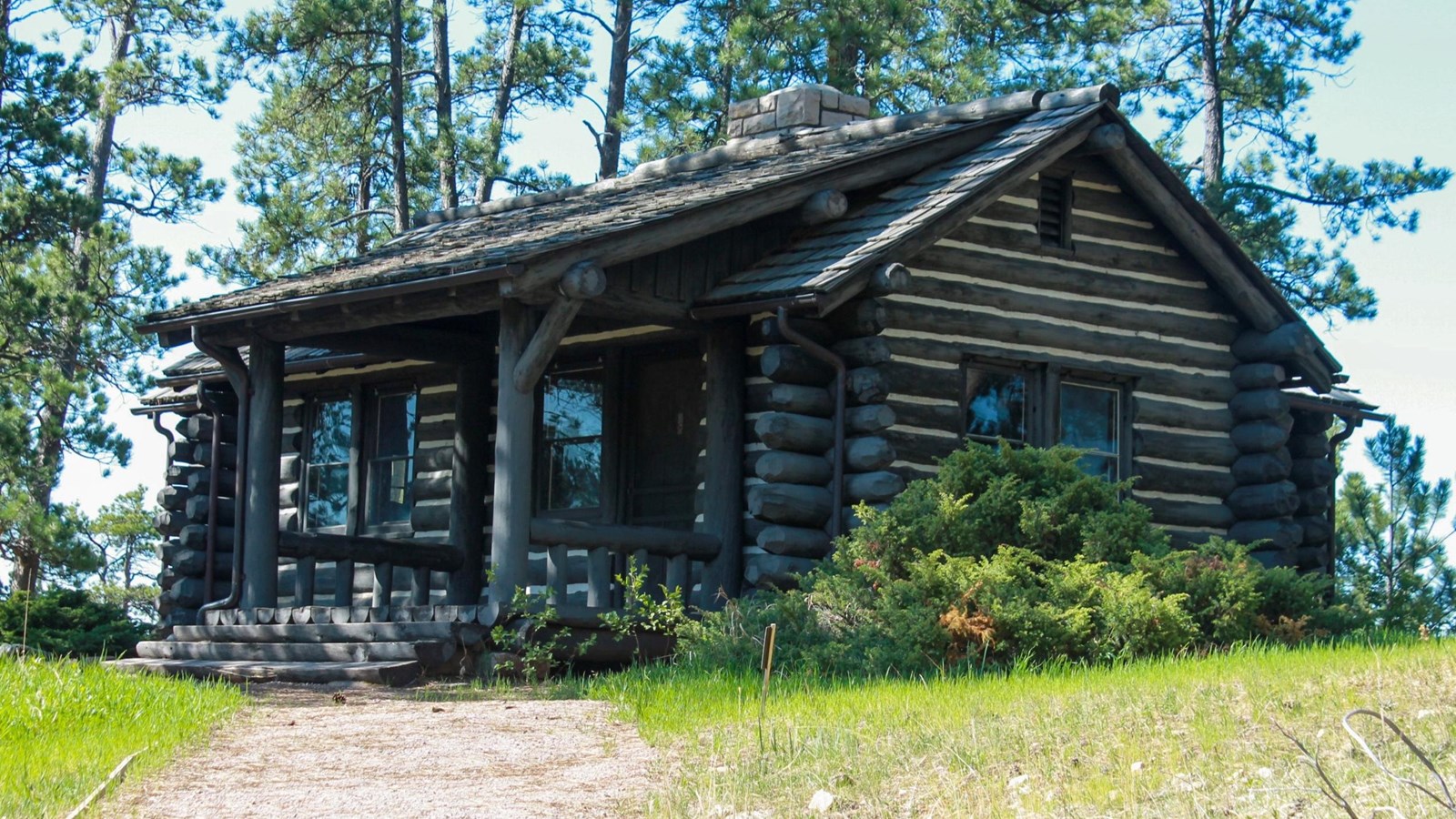The photograph captures an older wooden log cabin situated atop a gentle hill, framed by tall trees and a sky dappled with light blue hues and scattered clouds. A dirt pathway, commencing from the lower left corner of the image, winds its way through yellowish-green grass towards the cabin's wooden steps. The cabin, constructed primarily from long, dark brown or gray wood logs, features a distinctive notched log design, with the ends of the logs jutting out from the corners. The front of the cabin includes a porch area with wooden railings, supported by two sturdy logs, and a small set of steps leading to a main door. A brick chimney emerges from the cabin's roof, lending a rustic charm. The windows, which reflect a subtle blue light, punctuate the sides and front of the structure. To the right of the cabin, a large, green bush and smaller shrubs add a touch of wild greenery. The whole scene is bathed in the soft glow of daylight, highlighting the unkept grass patch in front of the cabin and the natural beauty of the surrounding landscape.